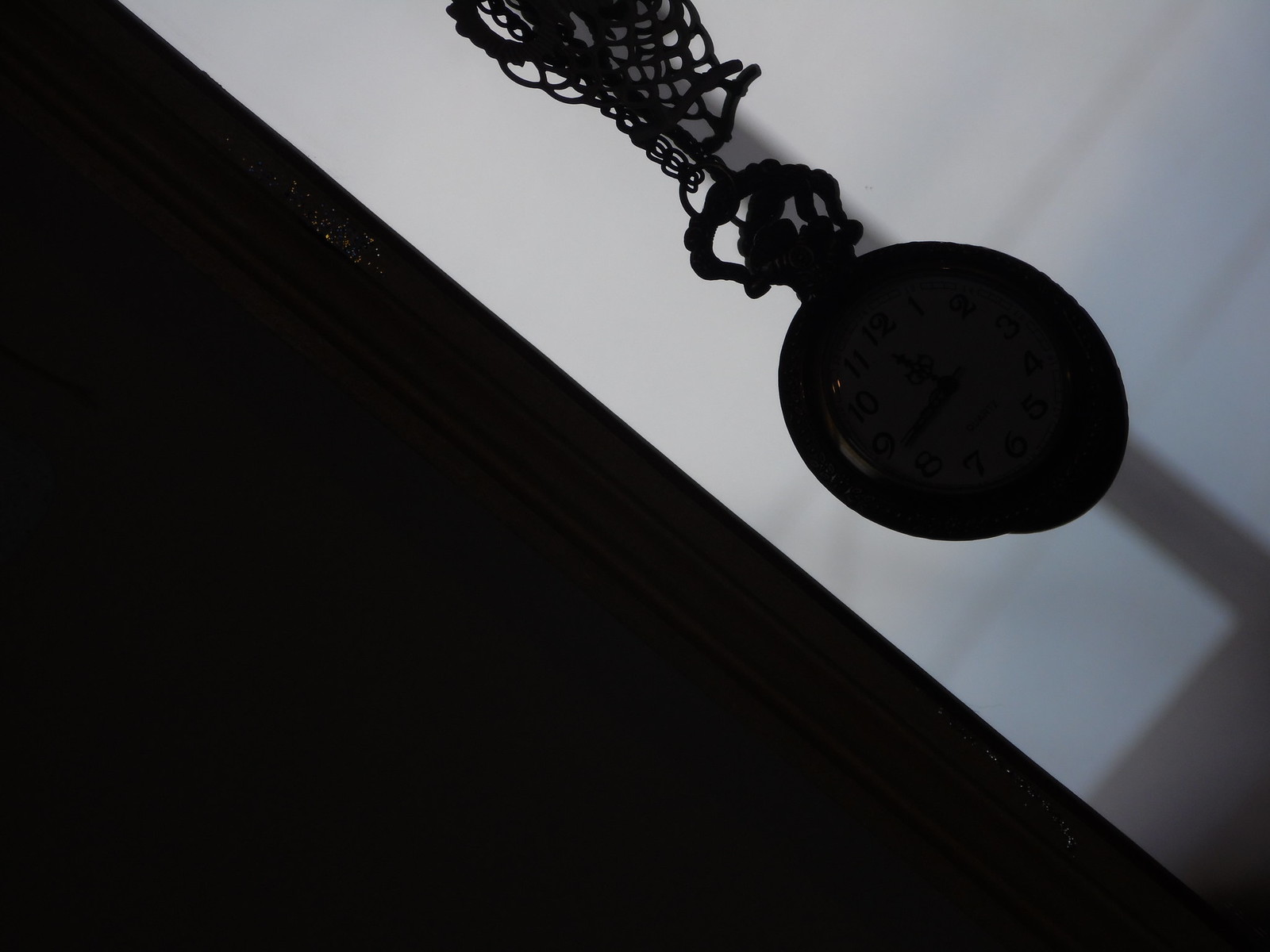This image features a clock hanging on a wall, captured from an unconventional angle. The viewer's perspective makes the wall appear to be the ceiling, with another wall to the left side of the image seemingly slanted. This creates an optical illusion of the left wall transitioning out of the shot while the right wall slopes downward, extending from the top-left corner to the bottom-right corner. The clock is positioned centrally in the image, descending straight from the top. It hangs at a slight angle on a white wall, contrasting with the left side of the image where the slanted wall exhibits a darker, whitish hue.